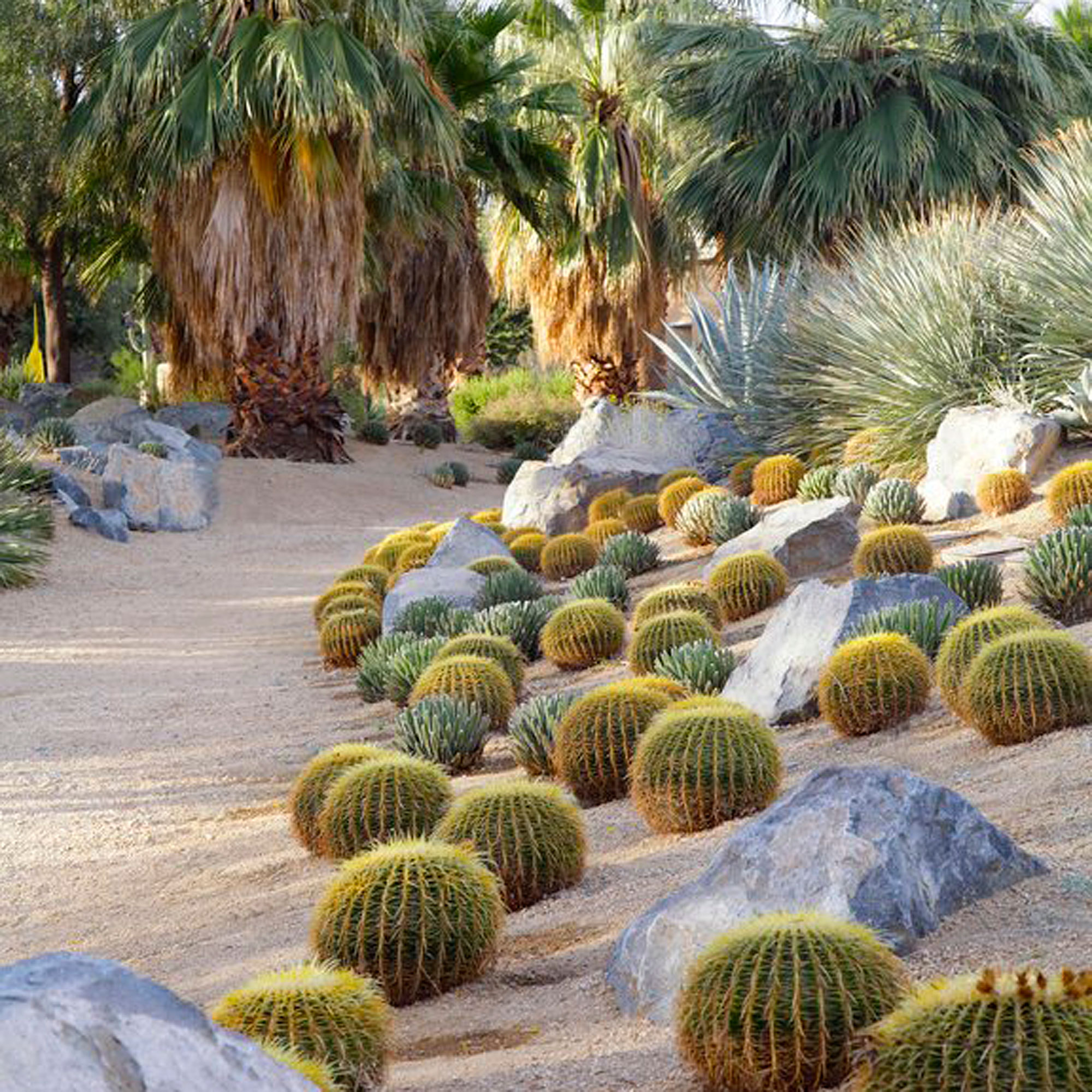This is a color photograph of a serene desert landscape, featuring a beautifully maintained sandy pathway with small gravel stones that curves in from the left and rounds towards the center. The pathway, appearing refined and evoking a vacation vibe, leads through a creatively landscaped area. On either side of the path, a diverse array of flora is artfully arranged, including numerous ball-shaped green cacti and other succulent-like plants. Scattered among the plants are large, jagged gray rocks partially buried in the sandy gravel. In the foreground, squat, almost circular ball-shaped cacti dominate the scene, while other spiky succulents and bushy plants intersperse the area. A tree line of short, chunky palm trees frames the scene, with a large palm tree visible in the background and others positioned towards the far right of the image. This photograph, devoid of any people, animals, buildings, or vehicles, exudes a tranquil and pristine desert garden atmosphere, perfectly capturing the essence of desert landscaping.